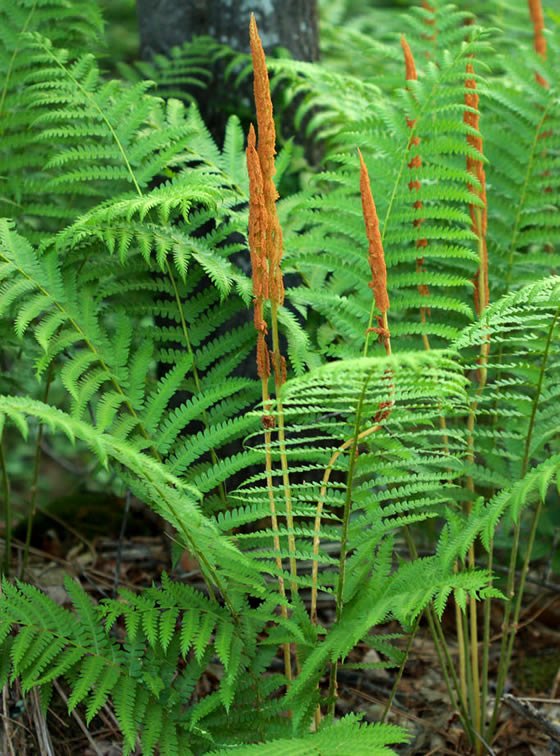This vibrant outdoor photograph captures a lush scene dominated by bright, healthy ferns, which are a vivid neon green, suggesting they have been flourishing for some time. The ferns, standing about a foot and a half tall, showcase their intricate long stems and smaller branching leaves, creating a thick, verdant backdrop. Amidst these ferns are clusters of burnt orange, cattail-like blooms that stand out prominently. There are two main blooms in the center, with the right one being significantly taller. This characteristic continues with a row of similar blooms extending toward the top right corner. Beneath the ferns, scattered dead leaves hint at their wild surroundings. Adding to the earthy ambiance, a sizable tree stump—indicating a forest setting—looms behind the fern cluster. The scene is bathed in bright light, possibly springtime, casting a lush and serene atmosphere overall.